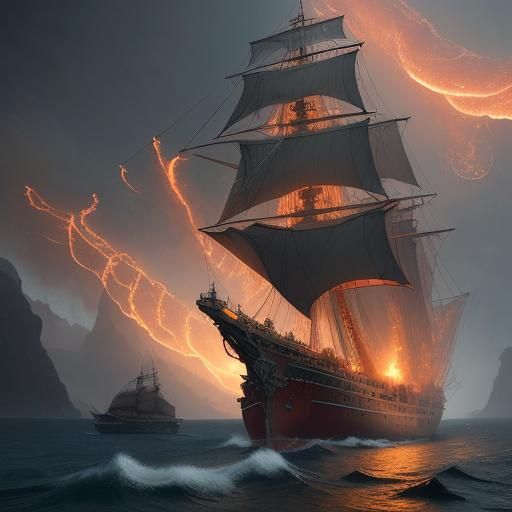The image depicts a dramatic scene centered around a large, old-timey pirate ship with an ominous atmosphere. The ship, dark red with brown wooden details, features four towering levels of white sails attached to a central mast. The sails reach almost to the top of the image, giving the ship a grand and imposing presence. The sky above is dark and gloomy, filled with blackish clouds and streaks of bright orange lightning, likely reflecting the setting or rising sun. The lightning appears to be emanating from the top of the ship’s mast and surrounding sails, adding an electrifying intensity to the scene.

On the left side of the main ship, in the distance, is a much smaller vessel, almost resembling a tiny yacht in comparison. The water below is dark and choppy, with visible white-capped waves, reflecting the turbulence of the stormy weather. In the background, the silhouette of rocky mountains can be seen on the left, adding further drama to the landscape. The bottom right corner of the painting captures the bright, orange reflection of the sun on the water, contrasting with the overall dark tone of the scene and highlighting the rough texture of the sea. Small figures can be spotted on the deck of the main ship, underlining its grand scale.